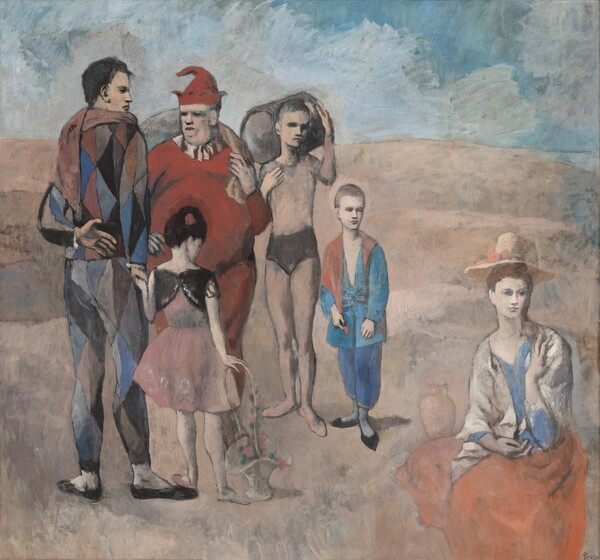This is a vintage painting, possibly done in acrylic, watercolor, or oil, of a group of people standing and sitting in an open, barren field under a mostly cloudy sky with hints of blue. The colors are muted and dark, lending a somber tone to the scene. In the bottom right corner, a woman sits, staring off into space. She is dressed in a red (or orange) skirt, a blue blouse, and a white shawl, topped with a hat adorned with flowers. To the left, a large man clad in an all-red, jester-like one-piece suit and pointy hat, resembling Santa Claus, stands with a white sack over his shoulder. Beside him, a tall man in a colorful argyle pattern outfit has his back to the viewer and his hand unusually placed behind it. A young girl in a pink ballet dress with a tiny vest and a flower in her hair holds a high-handled basket with flowers, standing near the man in argyle. Further to the left, a boy in brown underwear hoists a barrel over his shoulder, while another young boy next to him wears pointy ballet shoes, a blue blazer, and puffy pants. These figures, oddly grouped together, create a surreal, almost theatrical tableau.